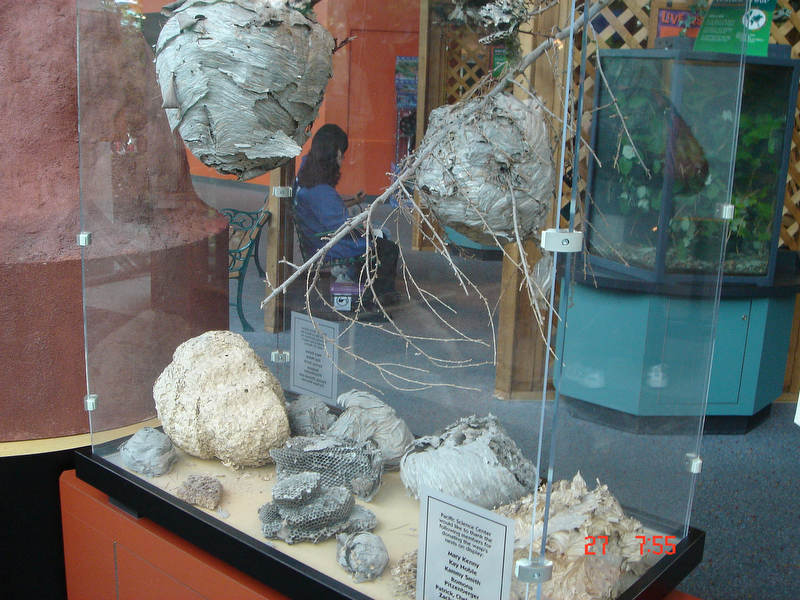The image depicts a wide rectangular display at a zoo or museum, featuring an orange wooden platform that extends diagonally from the center bottom and is cut off at the lower edge. Resting on this platform is a glass case with a black metal base, showcasing a sandy surface strewn with a variety of scaly, beige, silver, and gray objects resembling wasp or beehive nests. These nests are arranged in at least five or six distinct types, including some attached to sticks and others scattered on the ground. A white sticker with unreadable text is affixed to the glass case's front. In the background, the area is carpeted in gray, and a woman with long dark brown hair, wearing a blue sweatshirt, is seated on a nearby bench.